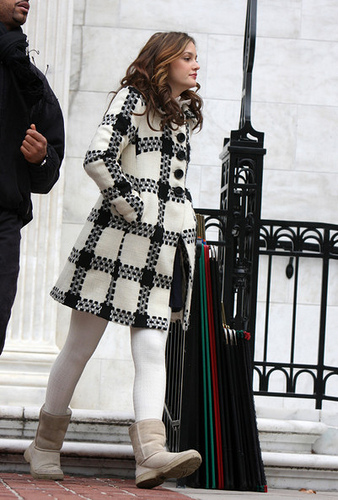In this image, a celebrity with slightly curly brown hair, highlighted to give a wavy effect, stands outside in front of a white stone building that could be a mansion or an older establishment. She is wearing a stylish outfit composed of a long, white and black checkered jacket with large black buttons, white leggings, and grayish-brown boots, reflecting a blend of cotton and polyester for warmth. She has makeup on and has clearly invested in her appearance. To her left, partially cut off in the image, stands an African American security guard dressed entirely in black, including a jacket and pants. He has a wristwatch on his left wrist and appears to have a walkie-talkie attached to his jacket. The setting features a black railing, a light post, and nearby steps on a red brick surface, adding depth to the scene.1